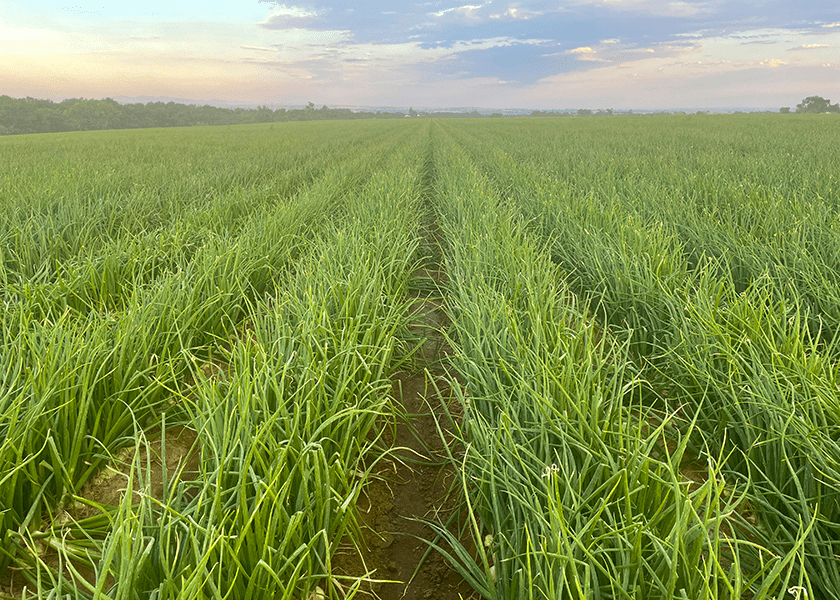The image depicts a vast agricultural field stretching towards the horizon, covered in orderly furrows brimming with dark green, vibrant plants resembling tall blades of grass, likely onions. Each plant, about a foot to a foot and a half long, shows the white bulbs just peeking out from the brown, slightly muddy soil, while their slender stalks appear ready to flower, indicating harvesting time is near. Despite the organized rows, the plants give a slightly unruly and untamed impression. In the background, a few dark green trees or possibly a mountainous region enhance the natural setting. Above, the sky is a light pinkish-blue with darker clouds hinting at impending rain, adding to the overall serene yet dynamic outdoor landscape.